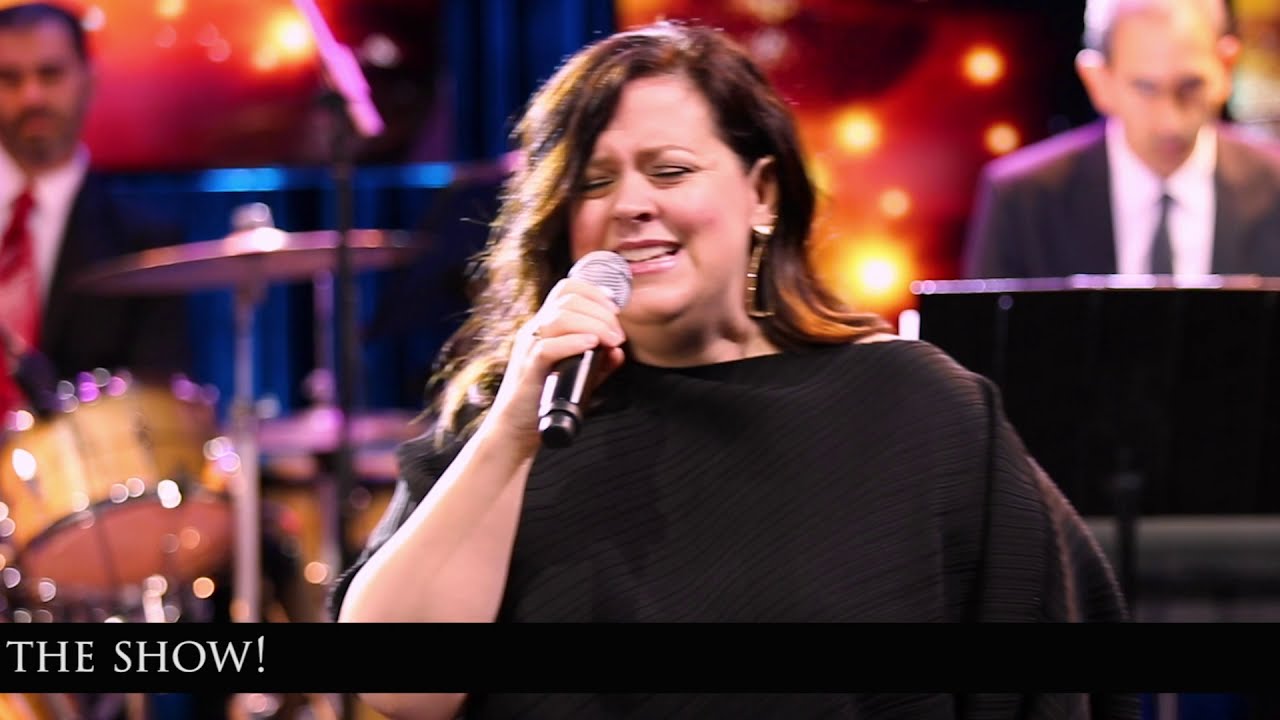In this image, a Caucasian woman with brown hair, styled to just below shoulder length and parted on the side, stands center stage. She's adorned with pink lipstick and large gold triangular dangling earrings. Clad in a black, silky blouse with sleeves reaching her elbows, she passionately sings into a microphone held in her right hand. Her eyes are closed, showing deep emotional engagement with the song. 

Behind her, the photo blurs slightly but reveals a well-dressed band. To the left, a drummer with brown skin, black hair, a beard and mustache, is visible. He is smartly dressed in a black suit with a white collared shirt and a red tie. On the right, there's a lighter-skinned man with a thinner build, playing the piano, also in a black suit with a white collared shirt and a black tie. 

The background glows with lights in yellow, orange, and blue hues, which emphasize the ambiance of a significant talent show, possibly resembling formats like Idols or America’s Got Talent. In the bottom left corner of the image, there's a black box with white text that reads "The Show," framing the scene as part of a formal televised event.